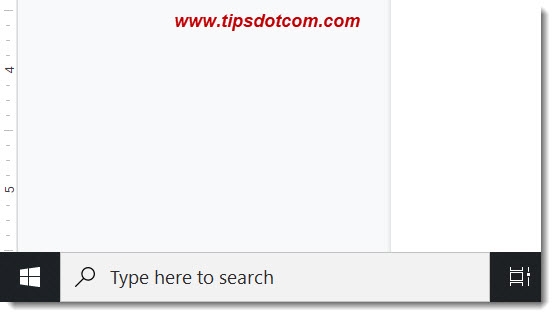This image features a screenshot of a word processing program on a Windows operating system, highlighting the bottom left corner of the application and the Windows toolbar.

On the left side of the image, a very slim, vertical ruler is displayed within the word processing document. The ruler includes precise markings: three ticks, the number 5, three more ticks, a larger tick, three smaller ticks, the number 4, three more ticks, and one larger tick.

To the right of the ruler is a large expanse of light gray negative space. Further to the right, the very edge of the document page is visible, characterized by its blank white appearance.

At the bottom of the screenshot lies the Windows toolbar, divided into several components. On the bottom left is a black square with a white Windows logo, composed of four squares arranged in a grid with a slight tilt to the left. This logo appears dimensional, with the left edge seeming farther away than the right.

Adjacent to the Windows logo is a light gray search box, featuring a black magnifying glass icon on the left and the text "Type here to search" on the right.

On the far right end of the toolbar, another black square is present, showcasing a white icon with three outlined rectangles stacked vertically. The top and bottom rectangles are only partially visible, giving the impression of half rectangles. Finally, to the right of this icon is a white line with a small white dot positioned about two-thirds up, presumably indicating some form of status or level.